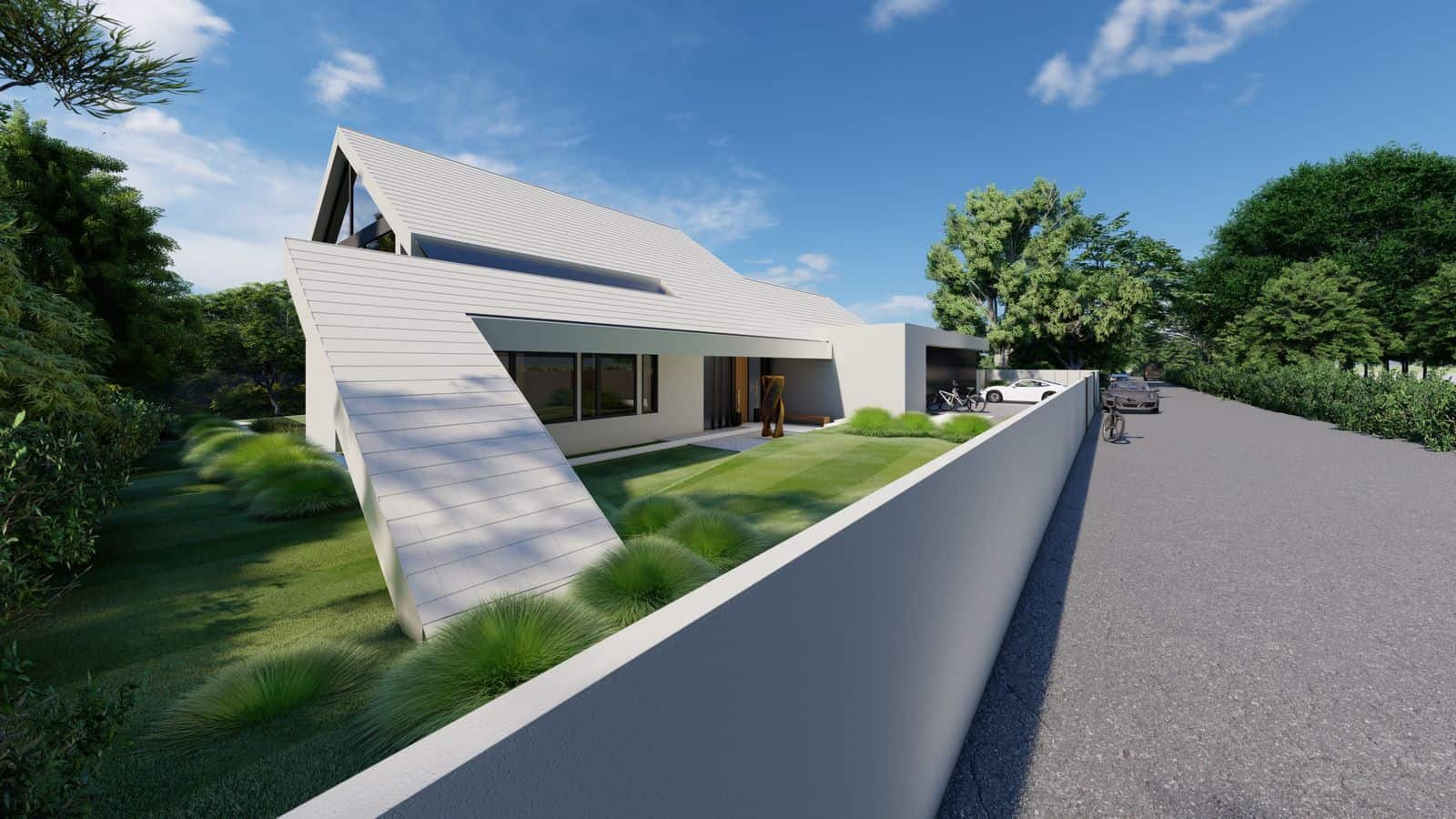This horizontally rectangular image, possibly a digital rendering, captures the sleek and futuristic design of a modern home that could also serve as a business office. The structure is elevated from the street by a white concrete wall, giving it a distinctive two-story appearance at the back while presenting a single-story front. The house, painted a crisp white, features a striking slanted roof that ascends towards the rear and then slopes downward on the left side. Large, expansive windows at the front enhance the modern aesthetic.

The property is lush with greenery, showcasing a well-maintained lawn and trees brimming with leaves on either side. To the right, there's a garage next to which a grey car is parked outside the fence, while inside the fence, a white car is visible. The driveway also hosts a couple of bikes. The encompassing neighborhood scene includes a road to the far right, visible behind the white fence, and additional parked cars and bikes.

Above, a mostly clear blue sky with minimal clouds sets a serene backdrop to the vibrant, green landscape, emphasizing the house's contemporary and pristine look. The house's positioning slightly off-center to the left, combined with the lush surroundings and sophisticated design, makes it a standout feature in this idyllic setting.